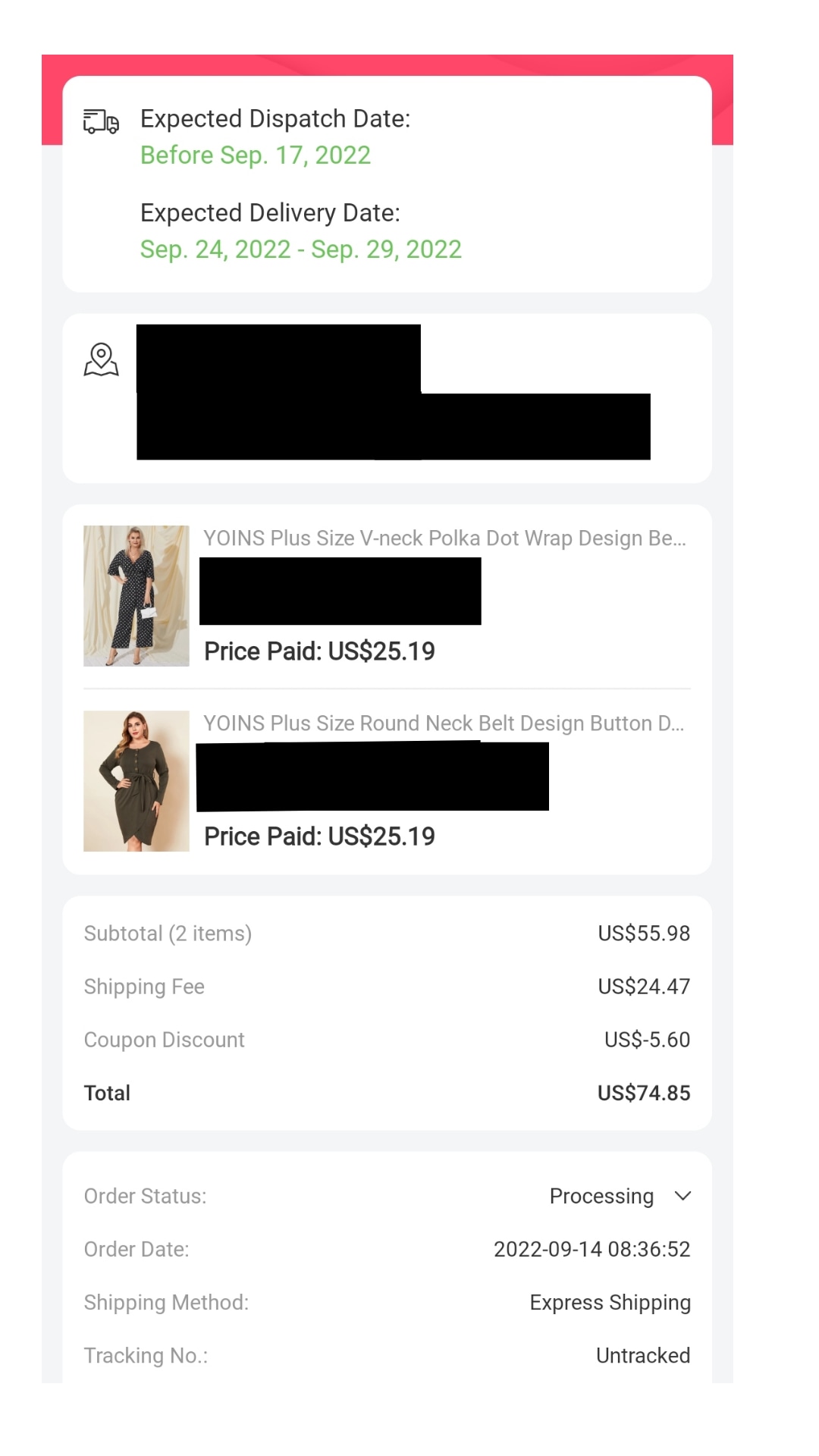The image displays an order confirmation document, prominently featuring a window with a red border at the top and some white space. The document appears to pertain to an online purchase from Yoins. 

At the center, green text indicates the expected discharge date as 'Before September 17, 2022,' and the expected delivery date as between 'September 24, 2022, to September 29, 2022.' An address is partially visible in black and white, identifying the recipient.

The document further lists two purchased items:
1. A "Yoins Plus Size V-Neck Polka Dot Wrap Design B," priced at $25.19.
2. A "Yoins Plus Size Round Neck Belt Design Button T," priced at $25.25.

The total sum for the two items is $50.44. Additional costs include a shipping fee of $24.47. A coupon discount of $5.60 is applied, bringing the total order amount to $74.85.

Additional details include:
- Order Date: 2022/09/14 at 08:36:52
- Shipping Method: Express Shipping
- Tracking Number: On Track